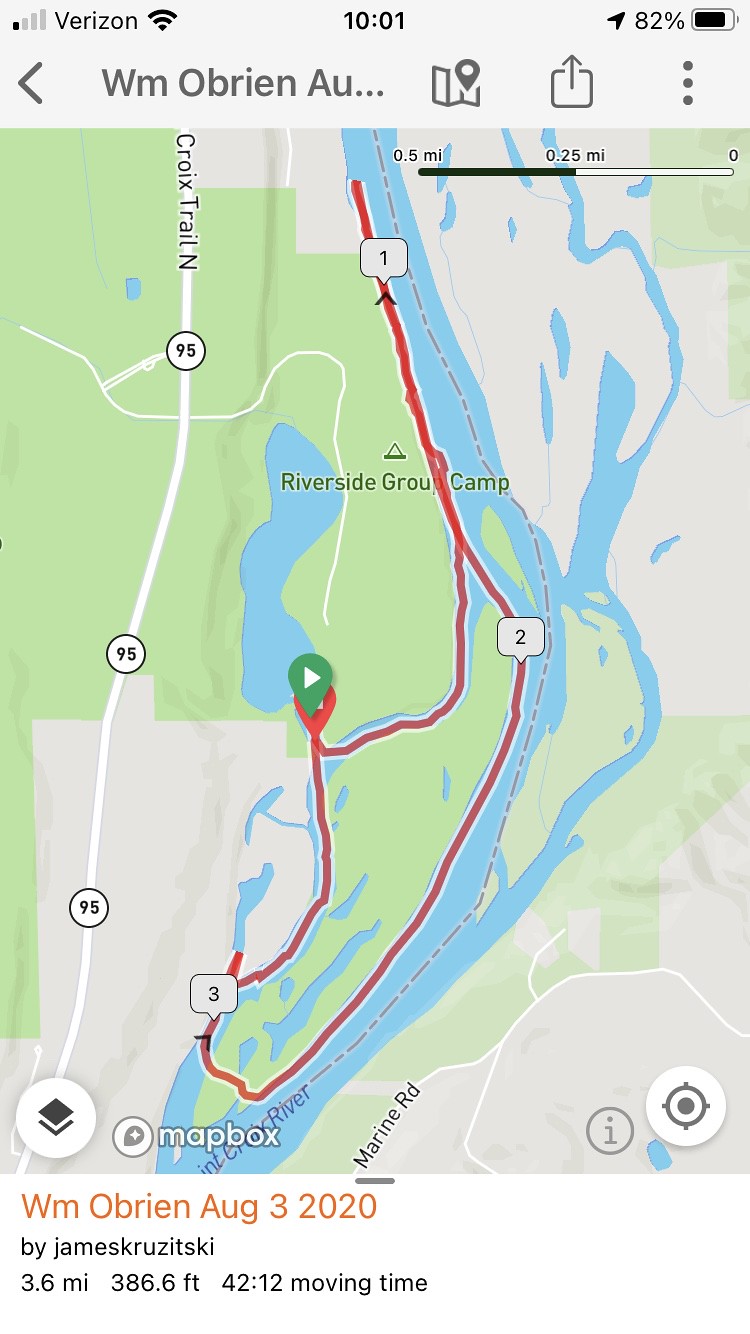This detailed caption integrates elements from all three descriptions, emphasizing shared and repeated details:

---

This image is a screenshot capturing a map from a cell phone display. At the top, the screen shows typical phone status information, indicating it is 10:01 AM, connected to Verizon with 82% battery life. Signal strength is indicated by one dark bar among four. Wi-Fi connectivity is also visible. Beneath this, a gray search banner displays "WM O'Brien AU," alongside icons for navigation, location, download, and options.

The dominant feature of the screenshot is a map, presenting a route in red. This route stretches diagonally, moving from the top-left towards the bottom-right, and includes sections where it splits into two converging lines with an arrow at the junction. The map also highlights major landmarks including the Quah Trail (labeled vertically as CROIX Trail N) and Marine Road. The map’s color scheme is detailed with green for land, blue for water, and red for the route. There are additional symbols and markers, such as white bubbles containing the number '95' along the trail path.

At the bottom of the screenshot, there is a textual overlay stating "William O'Brien, August 3, 2020," followed by "by James Skrzinski" (note the discrepancy in the last name spelling, which could be Skrzinski or Krusitzky). The final line details the nature of the movement: 3.6 miles, 386.6 feet elevation, and a moving time of 42 minutes and 12 seconds. This information is presented on a white background, emphasizing the specific details of William O'Brien's journey on August 3, 2020.

---

This caption consolidates the repeated and most critical details from the three provided descriptions into a coherent, detailed narrative.